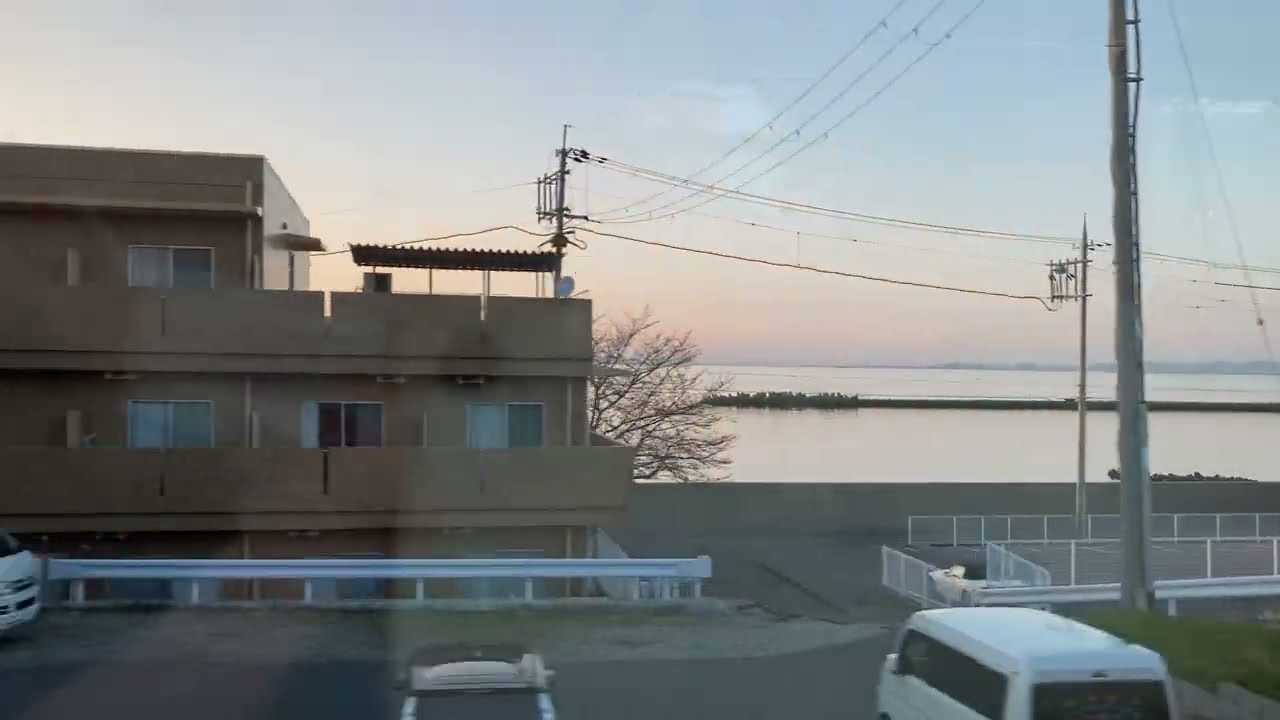In this photo, we see a serene scene of a large lake or bay extending into the distance, with a light brown apartment complex prominently featured in the foreground. The complex is built into the ground, lower than street level, and showcases several windows and balconies. To the left of the building, there's a concrete square structure with a balcony, a steel roof, and a satellite dish. Along the right side of the image, power lines stretch horizontally, supported by numerous electrical poles.

In the parking area at the bottom right, a white van is clearly visible. Further left, another darker van or truck is parked, and at the far left edge of the frame, the front of another white vehicle, likely a van, can be seen. A concrete platform separates the parking lot from the calm waters of the lake, and a barren tree can be spotted poking out from behind the apartment building.

The scene is bathed in the soft, pastel hues of either early morning or sunset, with the sky transitioning from a light blue at the top to a pinkish-orange near the horizon. In the far distance across the lake, a faint and blurry landmass is just visible. The entire composition exudes tranquility, with the still water and gentle lighting creating a peaceful atmosphere.